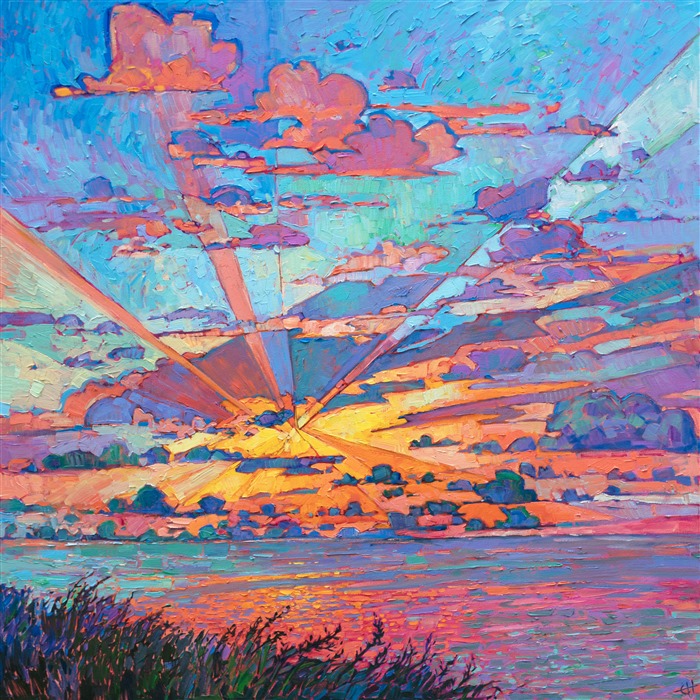In Erin Hansen's contemporary impressionistic painting "Radiant Light," a dramatic sunset fills the square canvas with a vibrant spectrum of colors. The artwork, at first glance, appears almost abstract due to its large, vivid blobs of pink, yellow, green, blue, and orange. Closer inspection reveals a dynamic scene segmented into geometric triangles, where the sky transitions from blue at the top to orange-red near the shoreline. Impasto brush strokes create rhythmic cloud patterns that radiate streaks of light from behind the clouds in bold, thick strokes. The sun, located near the bottom, casts beams across the painting, illuminating the landscape with an orangish-yellow tint. The water below mirrors the radiant sunset above, enhancing the reflective quality of the piece. In the foreground, on the left, grass and a few purple flowers add detail to the serene yet visually striking composition.